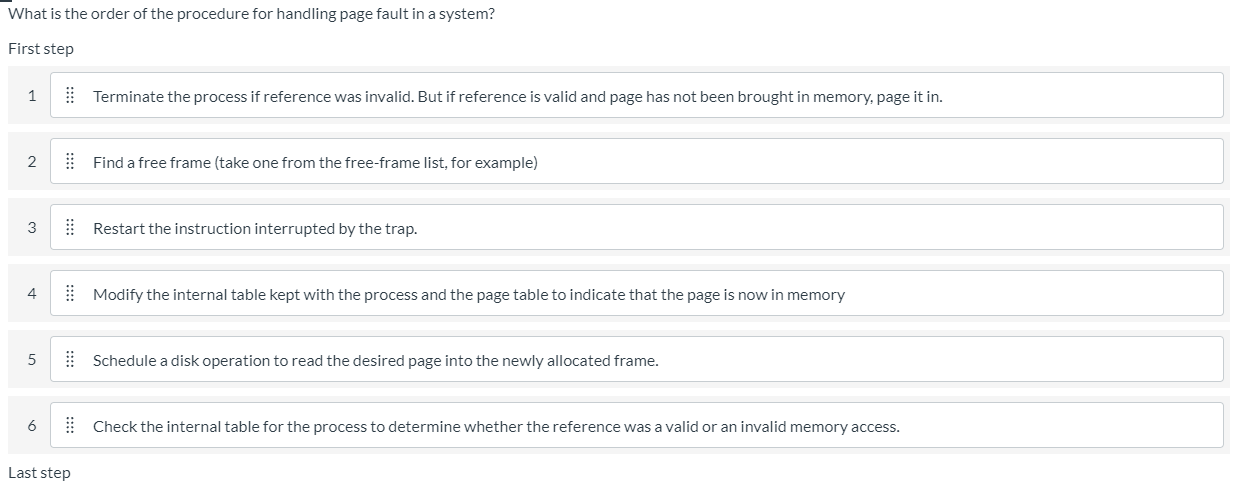In the top left corner of the image, a question is posed: "What is the order of the procedure for handling a page fault in a system?" Directly below this question is the label "First Step," followed by six sequentially numbered categories, each presented in individual rectangular boxes. The numbers 1 through 6 are displayed on a gray background, while the rectangular boxes are pure white. Each box contains detailed instructions for the procedural steps:

1. "Terminate the process if the reference was invalid. If the reference is valid but the page has not been loaded into memory, bring the page into memory."
2. "Find a free frame, such as selecting one from the free frame list."
3. "Restart the instruction that was interrupted by the trap."
4. "Modify the internal table kept with the process and the page table to indicate that the page is now in memory."
5. "Schedule a disk operation to read the intended page into the newly allocated free frame."
6. "Check the internal table of the process to ascertain whether the memory reference was valid or invalid."

Each step is meticulously detailed, guiding the viewer through the sequence of handling a page fault.